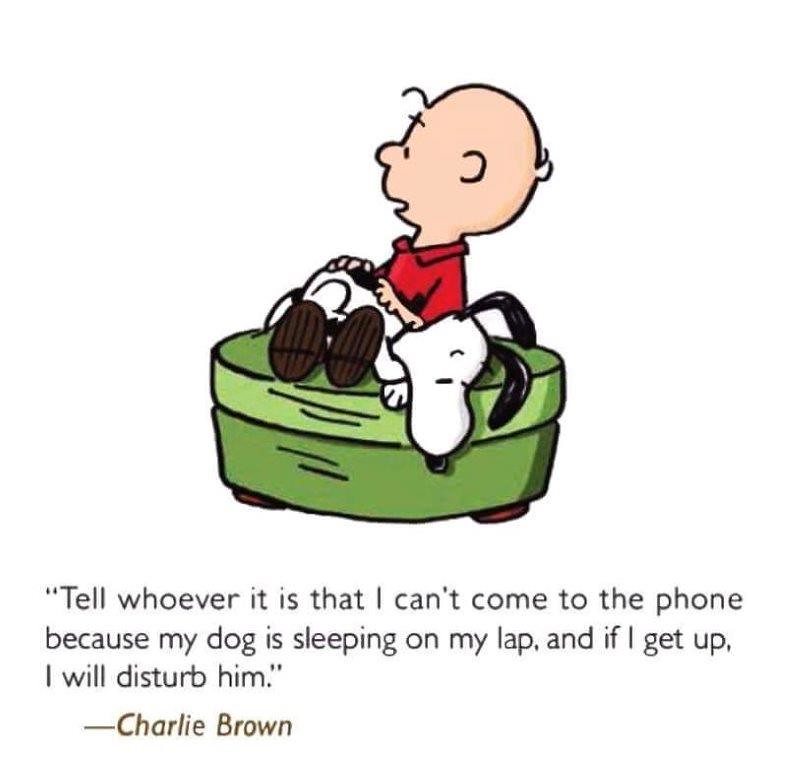In this detailed cartoon panel image, we see Charlie Brown from the renowned Peanuts series, standing beside a light green, two-tiered footstool. Charlie, wearing his iconic red shirt with a black zigzag stripe and brown shoes, gently pets Snoopy, his beloved white dog with black ears. Snoopy is comfortably lying on top of the footstool, appearing quite content. The background of the image is a plain white, ensuring all attention is drawn to the touching moment between the boy and his dog.

At the bottom of the panel, there is a heartwarming quote in black font: "Tell whoever it is that I can't come to the phone because my dog is sleeping on my lap and if I get up, I'll disturb him." This quote is attributed to Charlie Brown, with his name elegantly written in a brownish italic font. This delightful scene captures the tender bond between Charlie Brown and Snoopy, resonating deeply with pet owners who cherish those quiet, undisturbed moments with their furry friends.